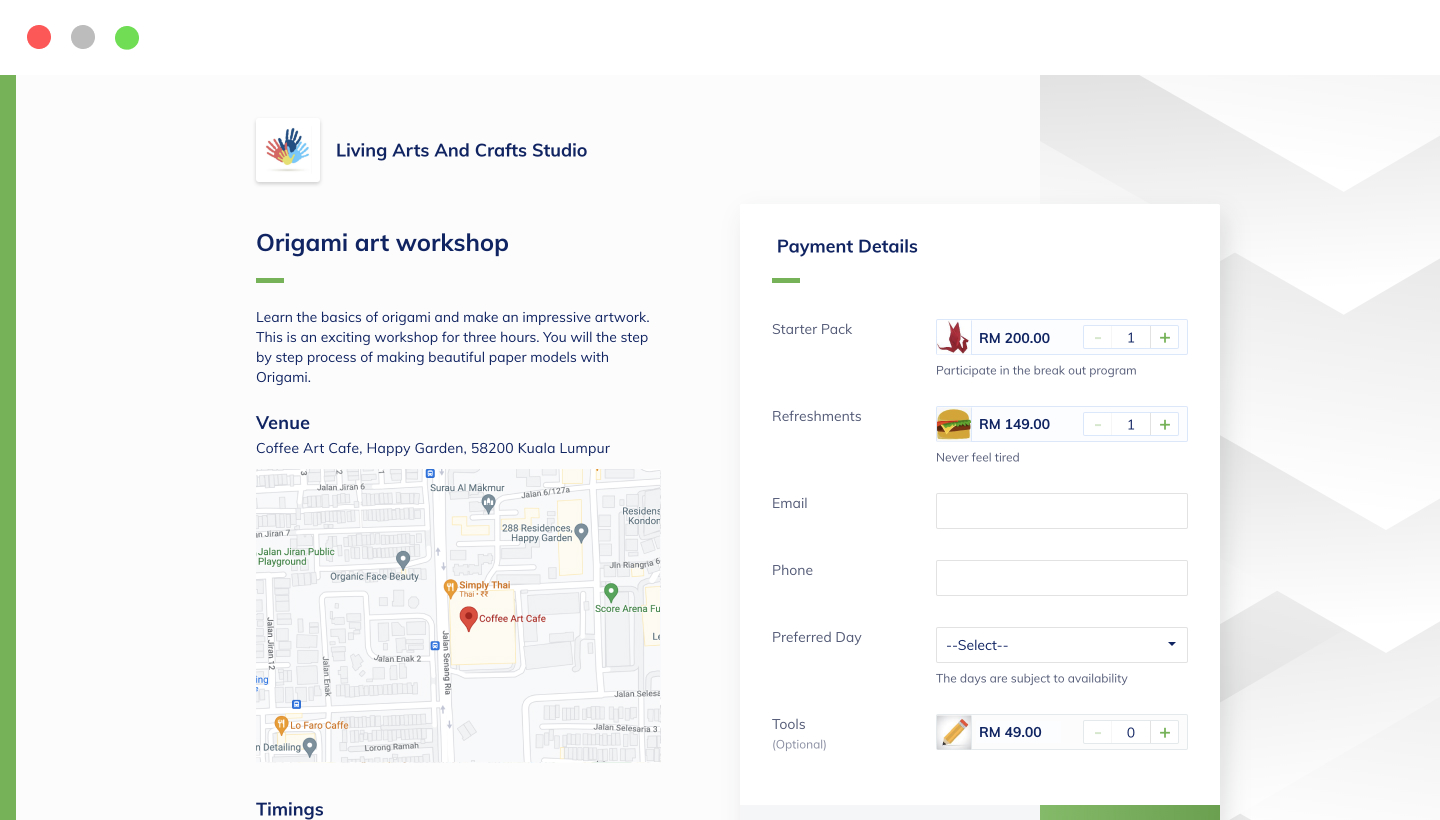**Desktop Screenshot on an Apple Device: Detailed Description**

The image captures a desktop screenshot on an Apple device, identifiable by the distinct program icons featuring the familiar "traffic light" buttons on the top left corner, though notably, the yellow button is replaced with a gray circle.

**Left Side:**
- A prominent green rectangle can be seen to the left of the screen.

**Right Side:**
- The right side showcases a gradient gray triangle mountain design.
- An icon representing a white square with multi-colored hands in yellow, orange-red, dark blue, and light blue is visible. Below the icon is the text "Living Arts and Craft Studio, Origami Art Workshop" with a partial green underline.
- Additional text in bluish-black reads: "Learn the basics of origami and make an impressive artwork. This is an exciting workshop for three hours. You will learn the step-by-step process of making beautiful paper models with origami. The venue is Coffee Art Cafe, Happy Garden, 58200 in Kuala Lumpur," alongside a map pinpointing the location.

**Right Section Details:**
- Below this, there is a section labeled "Payment Details" with a partial green underline.
  - **Starter Pack:** Shows an icon of what appears to be a red origami dragon with the price listed as RM200 (Malaysian Ringgit), and the quantity is set to plus one.
  - **Refreshment:** An icon of a burger is displayed with the price as RM149, with the quantity currently set to one. Above the burger, the text reads "Participate in the Breakout Room" and below it states "Never Feel Tired."
  - **Additional Fields:** There are fields for "Email" and "Phone," which are currently blank, and a drop-down list labeled “Preferred day,” noting that the days are subject to availability.
  - **Tools, Optional:** Shows an icon of a pencil, priced at RM49, though the quantity is not currently selected.

This detailed description illustrates that the screenshot likely involves a user looking to book an origami art workshop that includes options for purchasing food and tools, with fields available to complete the booking process.